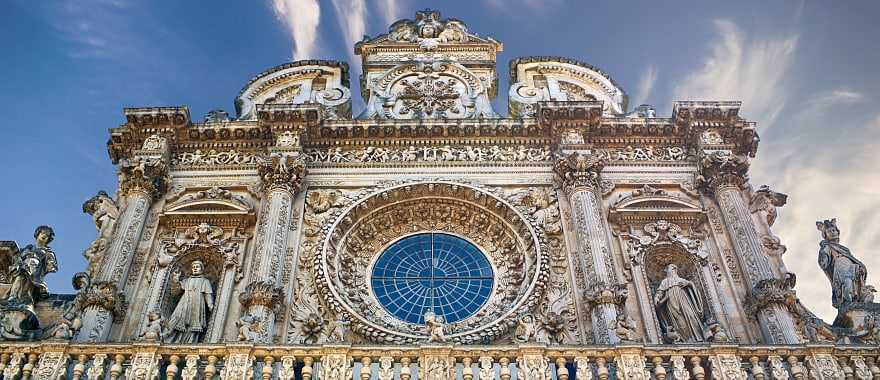This narrow, horizontal image captures the intricate upper portion of an ancient, ornately designed building, likely a church. The photo is taken from the ground, looking up, with the building dominating the scene. Set against a backdrop of a blue sky adorned with wispy white clouds, particularly concentrated to the right and just left of the center, the masonry structure showcases its historic grandeur.

At the center of the building's facade is a large, circular window, styled like an ornate bowl, featuring a blue core with a spider web-like pattern. Flanking this central element are four grand columns, each crowned with detailed sculptural figures. Beneath the roofline, smaller winged figures adorn the tops of these columns, adding to the building's elaborate decor.

Crowning the structure is an almost clock-like detail, displaying an angel poised above a heraldic shield. Atop the roof, a series of individual statues stand on a balustrade, depicting winged, helmeted figures dressed in flowing robes. Completing the scene, two alcoves house statues resembling friars, enhancing the ecclesiastical ambiance of the architectural masterpiece.